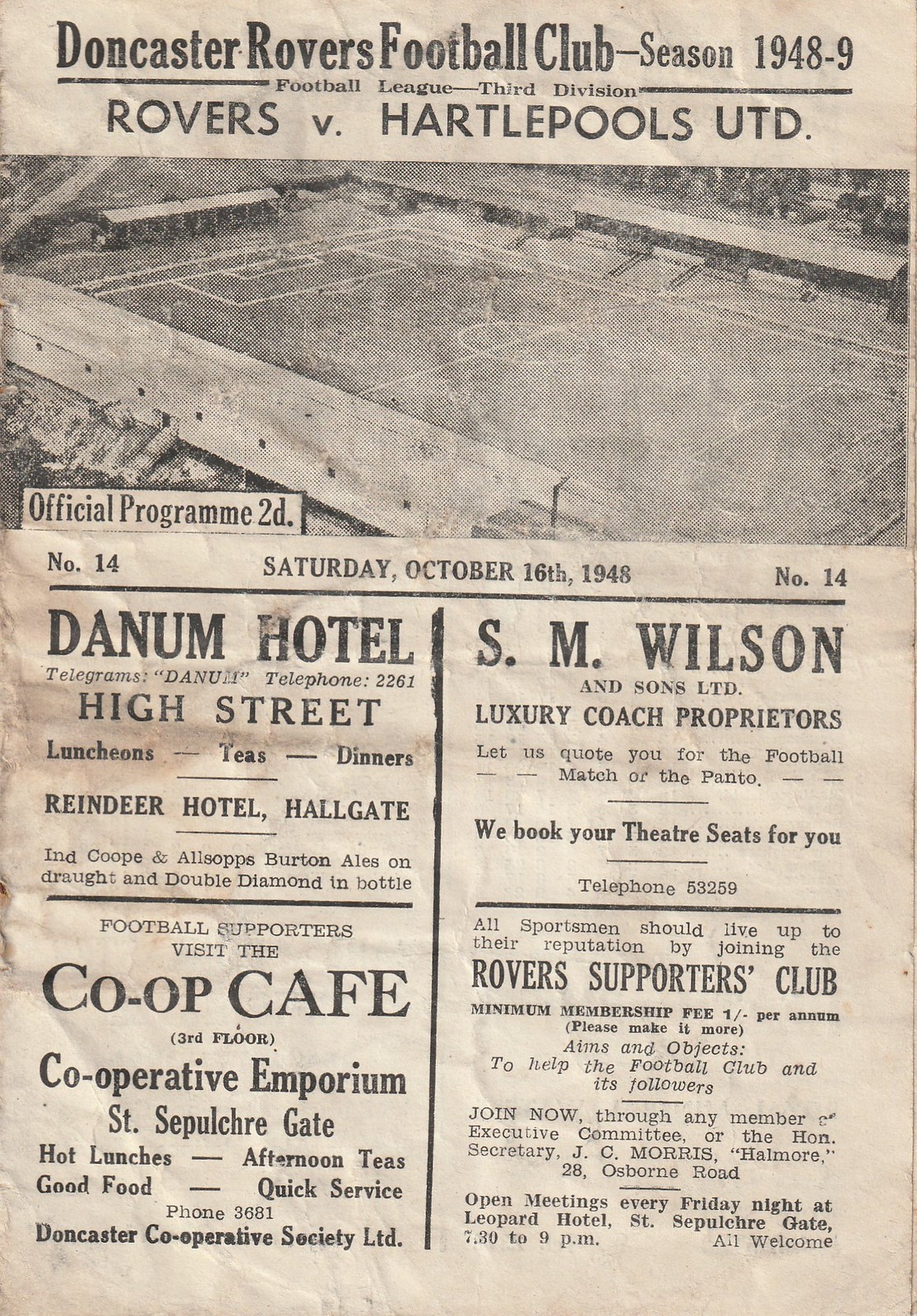This image is a vertically aligned rectangular photocopy of a worn and discolored newspaper article or booklet page, with a gray and white background. The headline at the top reads "Doncaster Rovers Football Club, Season 1948-9," followed by "Rovers vs. Hartlepools UTD." Beneath this, there is a very faded rectangular black and white picture of what seems to be a UK soccer field, suggesting that it is an official program for a soccer match. The image also indicates it was published for "Saturday, October 16th, 1948," marked as "Number 14" on both the right and left sides. The bottom section of the image contains four square advertisements. The upper left advertisement prominently features "Danum Hotel" in bold black letters, while the one to its right reads "S.M. Wilson." Both of these ads have additional smaller text underneath. The lower left corner showcases "Co-op Cafe," and the lower right corner advertises the "Rovers Supporters Club." The overall aesthetic of the page and its color palette, primarily tan, black, and various shades of gray, further emphasizes its vintage and historical nature.